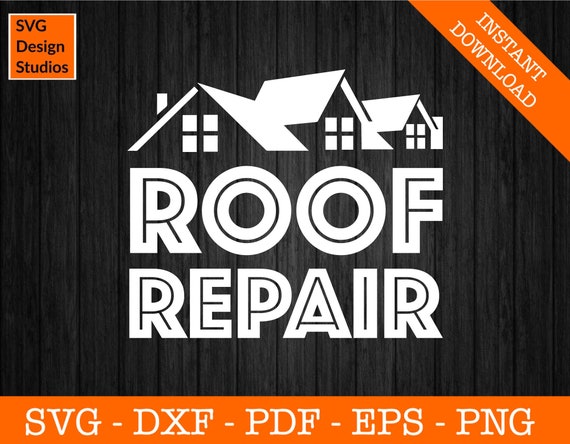This digital advertisement for "Roof Repair" features a striking visual design against a black background resembling painted wood panels. Central to the image is an illustration of three white roof silhouettes, each showcasing different angles and featuring elements like chimneys and windows, representing a large house. The bold white text, "Roof Repair," prominently adorns the middle of the graphic. In the upper right corner, an orange diagonal banner declares "Instant Download" in white letters, indicating the immediacy of the service. The top left corner features a small orange square with a black outline housing the logo "SVG Design Studios." An additional horizontal orange banner runs across the bottom of the image, listing file formats available for download: "SVG, DXF, PDF, EPS, PNG" in large, clear white font. This advertisement suggests a customizable, downloadable design tailored for roofing companies.